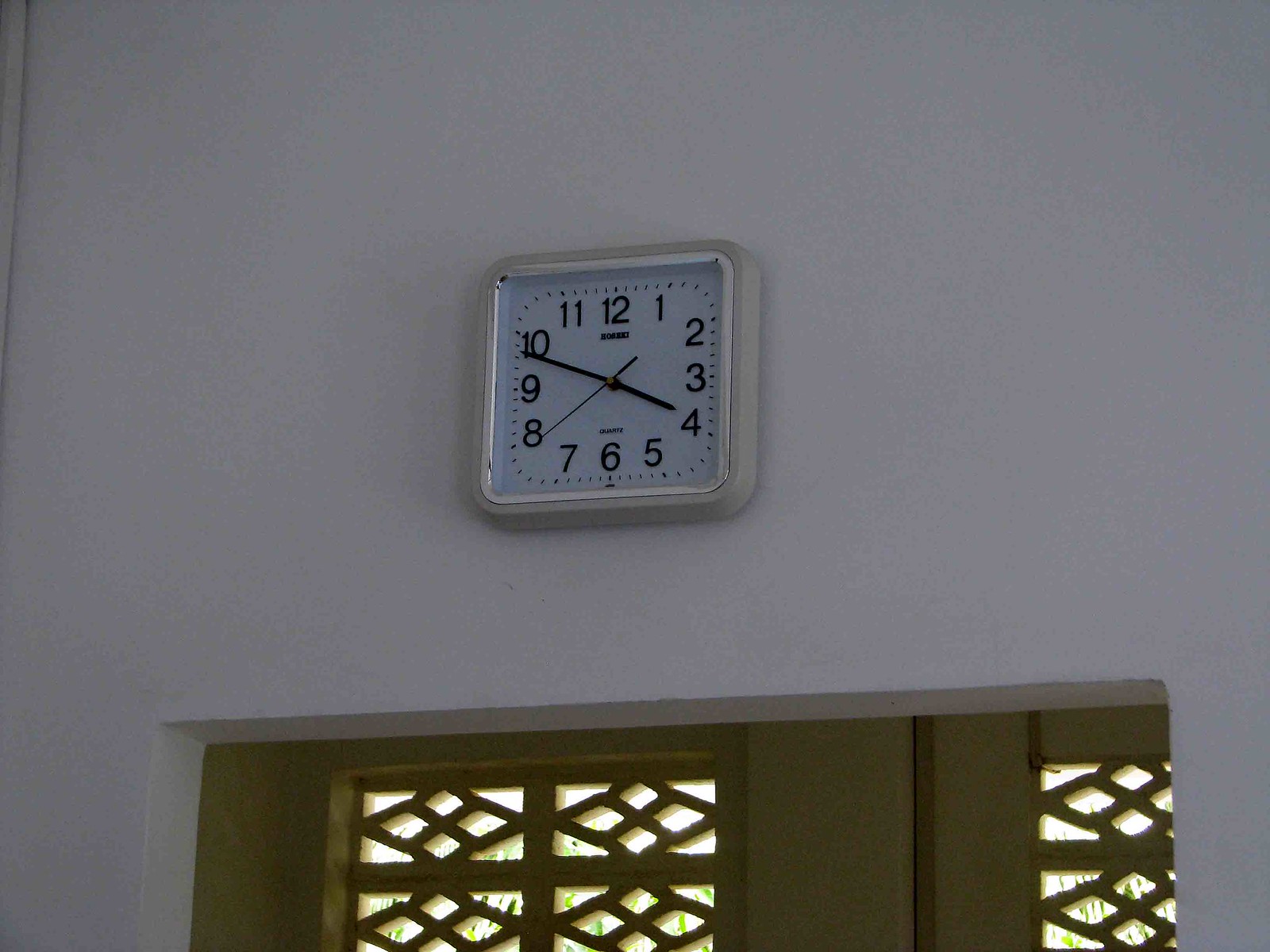This indoor photograph captures a minimalist analog clock mounted on a pristine white wall. The clock features a rounded square frame that appears in an off-white or light grey tone, contrasting with its very white face. The clock’s design is straightforward, with black numbers from 1 to 12 and black hands, including a second hand currently pointing near the 8, indicating the time is 3:48. The face also includes small dots encircling each number. Below the clock, a stylized wooden door with triangle patterns and possible cross and flower designs is visible, suggesting a church-like design. The scene is well-lit, potentially by sunlight, enhancing the simplicity and clarity of the wall and clock.